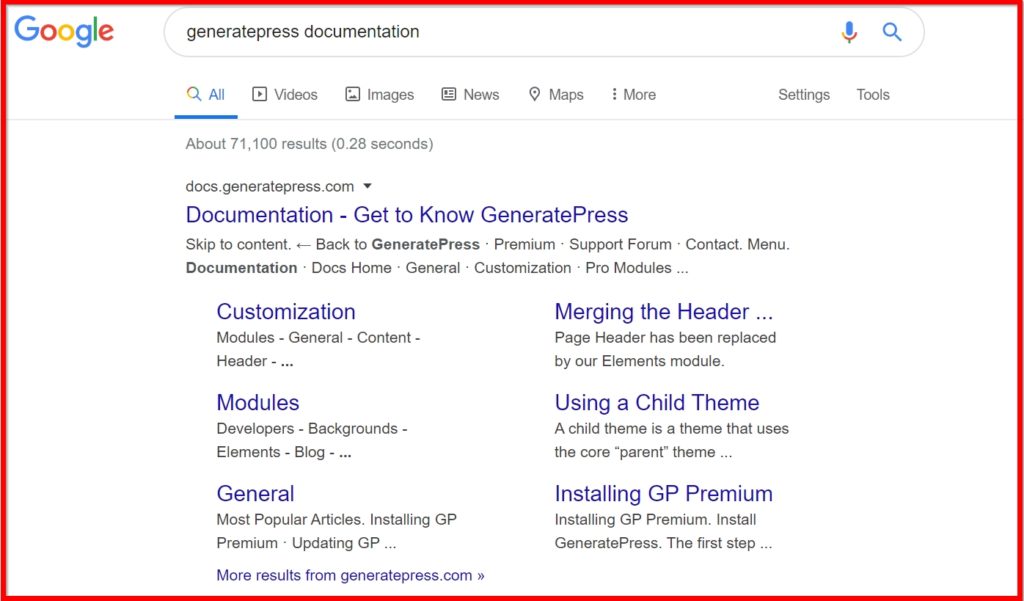The image is a horizontal screenshot of a Google search results page, framed by a prominent red border. The page has a clean white background with text in varying hues of purple, blue, and black. In the upper left corner, the colorful Google logo is visible, followed by the search bar to its right, containing the query "GeneratePress documentation."

The search results indicate that the "All" tab is selected, highlighted in blue. The primary search result is titled "Documentation: Get to Know GeneratePress," displayed in purple text. Below the title, there's smaller text providing additional details.

Further down, various categories and topics related to GeneratePress are listed, including "Customization," "Modules," "General," "Merging the Header," "Using a Child Theme," and "Installing GP Premium."

Additionally, there is more black text beneath the main documentation heading, offering quick links such as "Skip to Content," "Back to GeneratePress," "Premium," "Support Forum," "Contact," "Menu," and navigational options like "Documentation," "Docs Home," "General," "Customization," and "Pro Modules."